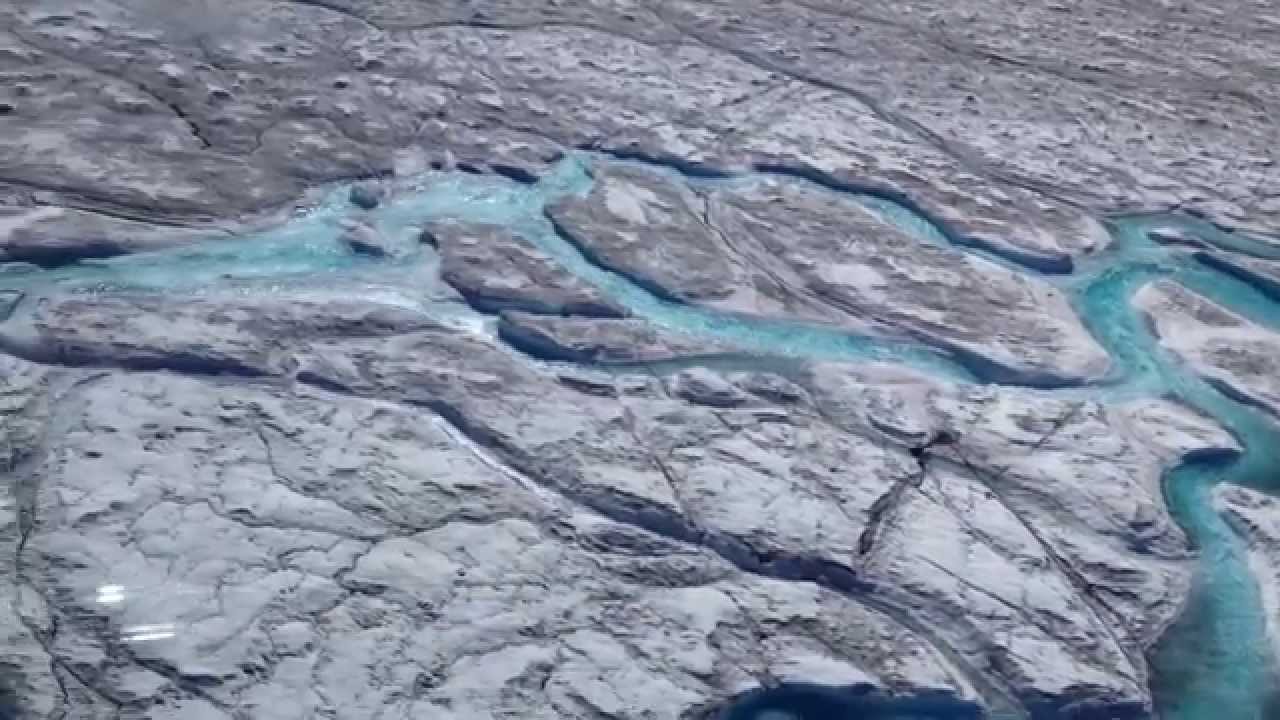The image captures an expansive, flat, and smooth gray rock formation outdoors, resembling an island or landmass with oceanic features. The rock surface, which occupies the majority of the frame, appears to have been gradually smoothed and shaped by water over time. This landmass is crisscrossed with crevices, through which flows a meandering body of turquoise, aquamarine blue water, giving the impression of a fluid yet somewhat blurred motion. The photograph seems to have been taken from an elevated, aerial perspective, looking down at the scene. Despite the somewhat photographic quality of a video still, the blue water cuts horizontally across the image and curves intricately through the rock's natural striations, enhancing the dynamic yet serene atmosphere. No people or animals are present, allowing the natural interaction between rock and water to be the focal point.